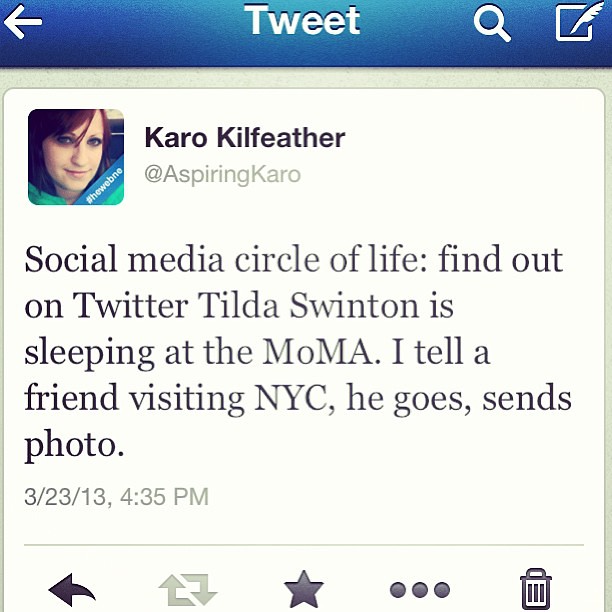The image depicts a screenshot of a tweet viewed on a mobile interface, dominated by a blue bar at the top. On the top left, there is a bold left arrow icon, with the white title "Tweets" in the center and a magnifying glass icon for search on the right. Next to the search icon is a square icon with rounded edges containing a feather quill, symbolizing the compose tweet function.

Beneath this bar, there is a white rectangular card featuring a profile image of a smiling woman with red hair in the top left corner. To the right of the profile image, the name "Karo Kilfeather" appears in bold black text, accompanied by the handle "@aspiringKaro" in light gray.

The tweet itself reads: "Social media circle of life; find out on Twitter: Tilda Swinton is sleeping at the MoMA. I tell a friend visiting NYC, he goes, sends photo." Below the tweet, light gray text indicates the date and time "3/23/13 at 4:35 p.m."

At the bottom of the card, a series of icons are displayed for interaction: a curved left arrow for reply, two arrows forming a square for retweet, a star for favorite, three dots for more options, and a trash can icon in the bottom right corner.